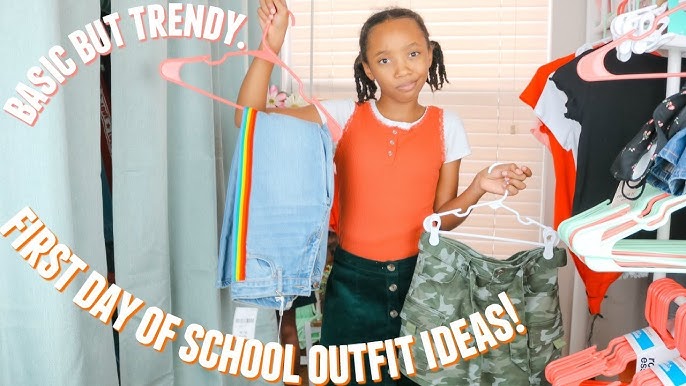The image features a young girl with dark skin, standing in front of a closet filled with various clothes hanging on a rod. She is wearing an orange tank top over a white t-shirt and black shorts. Holding a pair of bottoms in each hand, she displays a pair of light blue jeans with rainbow-colored accents on a pink hanger in her right hand and green camouflage cargo shorts on a white hanger in her left. The backdrop includes a window with peach-colored blinds. The caption on the image reads, "Basic but Trendy First Day of School Outfit Ideas." In addition, there are assorted colored hangers, mint green, salmon, and white, visible among the hanging clothes, enhancing the scene's vibrant and organized aesthetic.